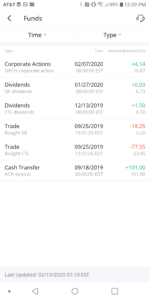The image portrays a smartphone screen with a low resolution, making some elements difficult to read. In the top-left corner, the status bar shows "AT&T" along with various icons. On the top-right, the time is displayed as "12:09 PM," with a battery icon indicating 99% charge. Below the status bar, the word "Funds" appears with a left-pointing arrow beside it. To the right, a headphone icon with a microphone is visible.

The interface is divided into two tabs: "Time" on the left and "Type" on the right. The main section of the screen lists various transactions and events. The details are as follows:

1. **Corporate Actions:** 
   - Date: 02/07/2020
   - Time: [Unreadable due to resolution]
   - Change: +4.14 (in green)

2. **Dividends:**
   - Date: 01/27/2020
   - Change: +0.03

3. **Dividends:**
   - Date: 12/13/2019
   - Change: +1.50

4. **Trade:**
   - Date: 09/25/2019
   - Change: -18.25 (in red)

5. **Trade:**
   - Date: Same as above (09/25/2019)
   - Change: -77.55 (in red)

6. **Cash Transfer:**
   - Date: 09/18/2019
   - Change: +101.00

Each entry includes a date, some in yellow text, with the corresponding financial change either in green (positive) or red (negative).